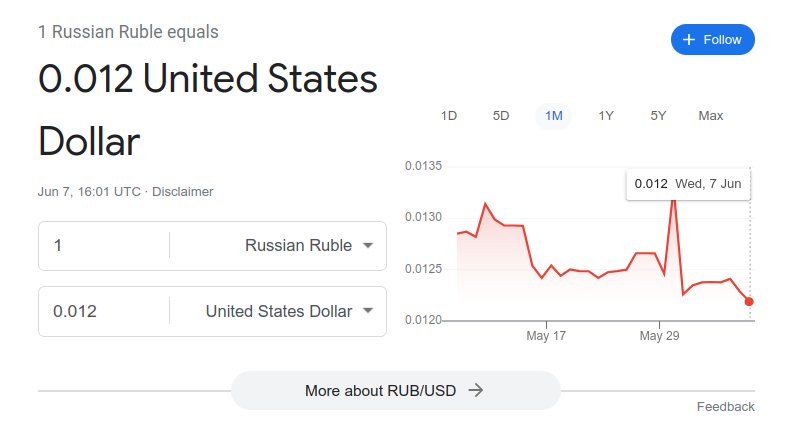The image displays a detailed representation of currency conversion from Russian rubles to United States dollars. At the top, written in grey, it states, "One Russian Ruble equals," followed by a prominent black bold text displaying "0.012 United States Dollar." In the top right corner, there is a dark blue oblong shape with a white plus sign and the word "Follow" written inside it.

Beneath the "United States Dollar" value, the text "June 7th, 1601 UTC - DISCLAIMER" is visible. Just below this, there are two boxes with drop-down menus on the right. The top box has "1" on the left, and the drop-down menu indicates "Russian Ruble." The bottom box has "0.012" on the left, and the drop-down menu indicates "United States Dollar."

To the right of these boxes, there is a graph. The y-axis of the graph ranges from "0.0120" to "0.0135." The x-axis shows a timeline from "May 17th" to "May 29th." In the top right corner of the graph, it displays "0.012 Wednesday, 7th June," and a red line spans across the graph horizontally from left to right, indicating a constant rate of 0.012.